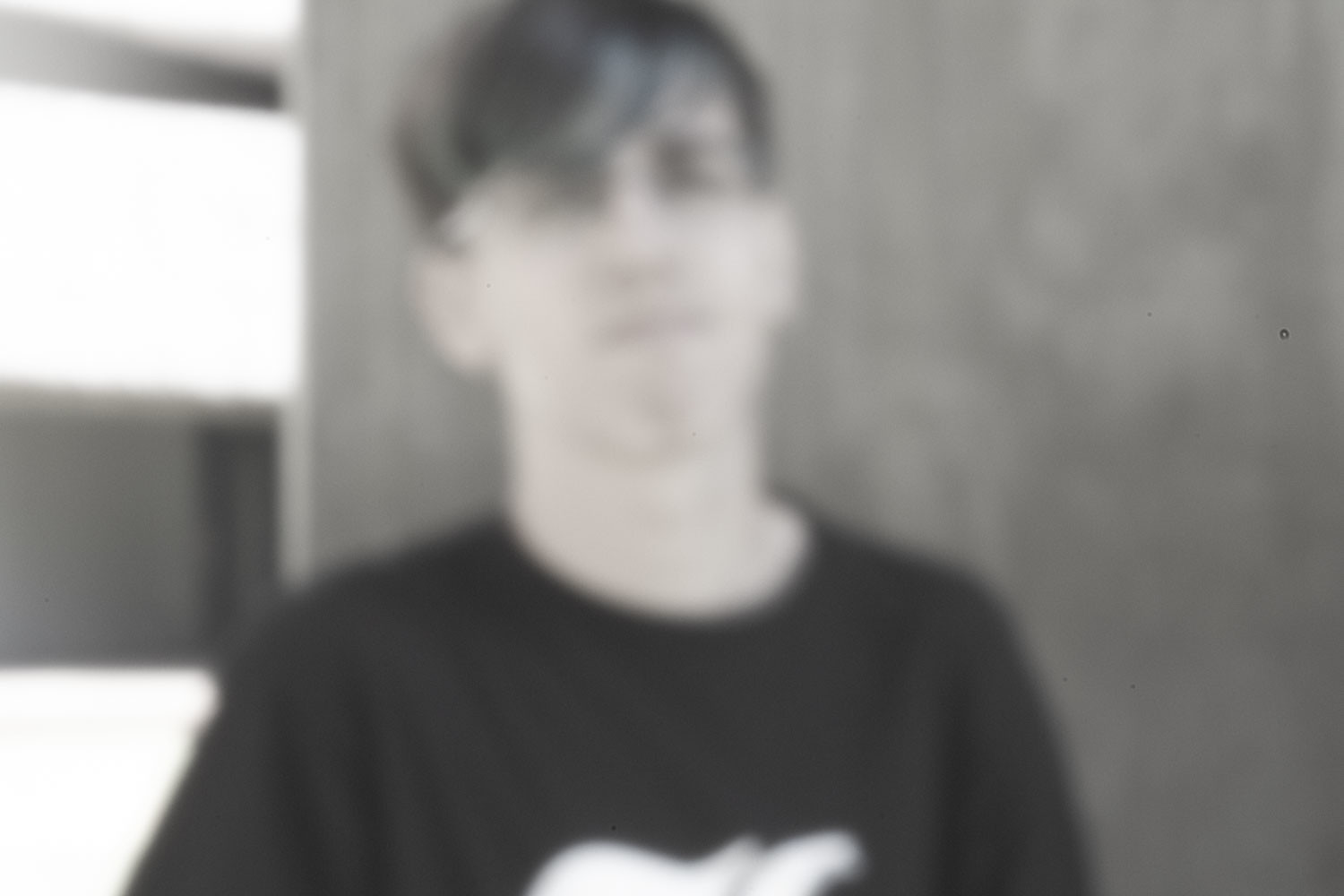A blurry black-and-white photograph features an ambiguous figure, likely a gentleman or a woman with short, dark hair that includes noticeable bangs. The hair is either pulled back or cut short. The entire image suffers from severe out-of-focus issues, rendering the foreground, the person, and the background indistinct. The individual stands before a wall that includes segmented window panels situated in the photograph's left corner. The person is dressed in a black T-shirt adorned with a partial white logo or design resembling the top of a guitar headstock.